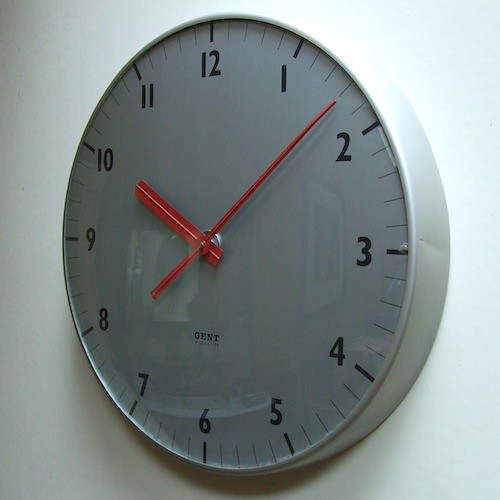Against a stark white background, a clock with a reflective face is mounted on a white wall. Light flares gracefully at the far-right edge of the image, casting an intriguing shine on the clock's surface. In the reflection on the clock's glass cover, a framed painting can be seen hanging on the right side of the wall. The clock is designed with black numerals from one to twelve and features small dash markers encircling its periphery. At its center, a pair of metallic silver hands is positioned, with the hour hand pointing towards the 10 and the minute hand resting between the 1 and 2. The serene yet sophisticated setup is subtly disrupted by the light flares, giving the scene a dynamic visual element.